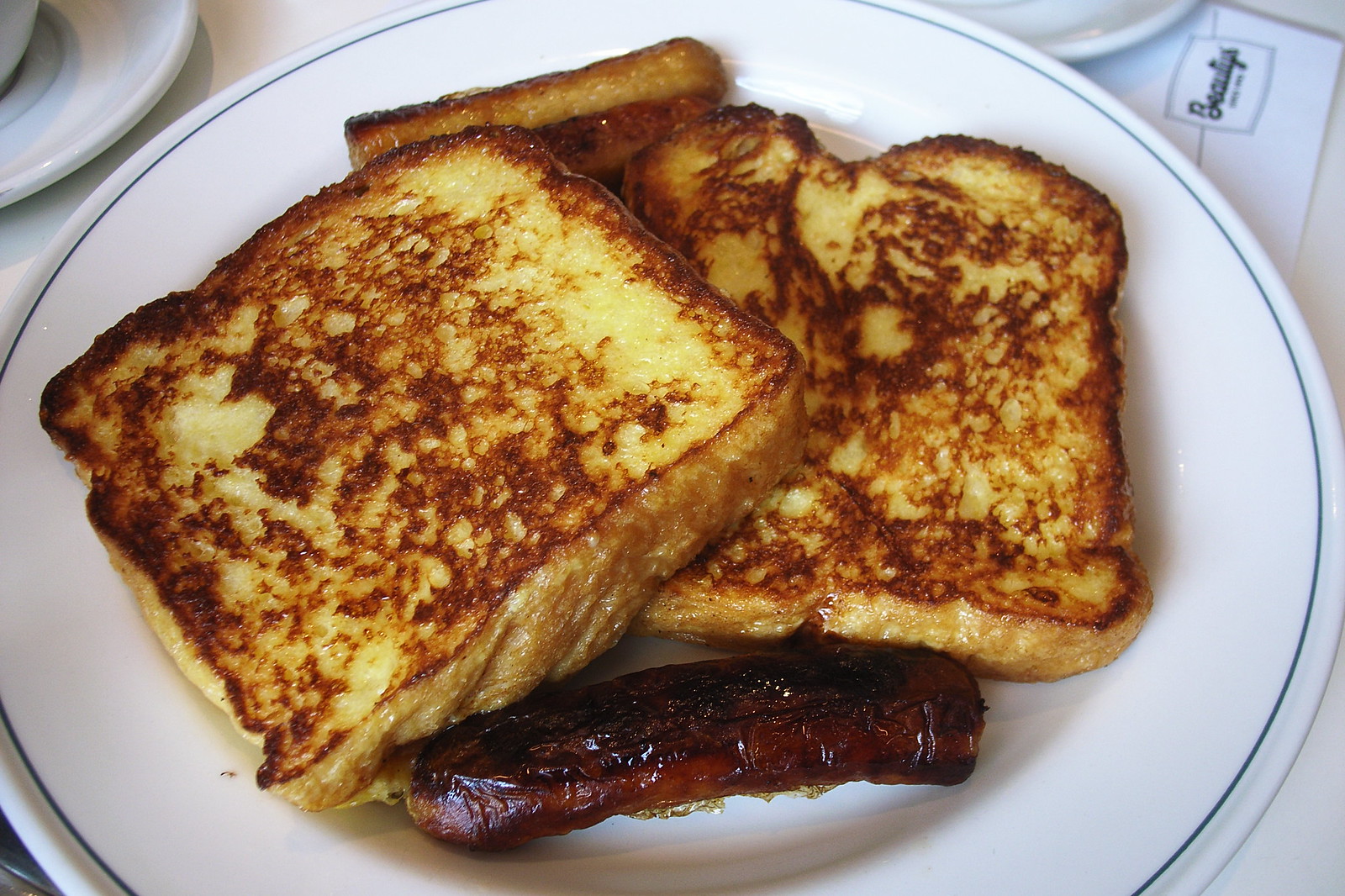The image captures a delectable plate of brioche French toast with sausage links arranged on a white plate featuring a thin bluish-black line around its rim. The French toast, consisting of two thick, buttery, and glossy slices, is positioned with one piece slightly overlapping the other. Crispy sausage links are placed at the top and bottom of the plate; the top sausage is lighter in color, while the bottom sausage is well-browned. The table setting includes a white tablecloth and additional, partially visible plates, suggesting a dining setting that might include a coffee cup and saucer at the top left corner. There's also a partially visible napkin on the right side featuring some unreadable text.